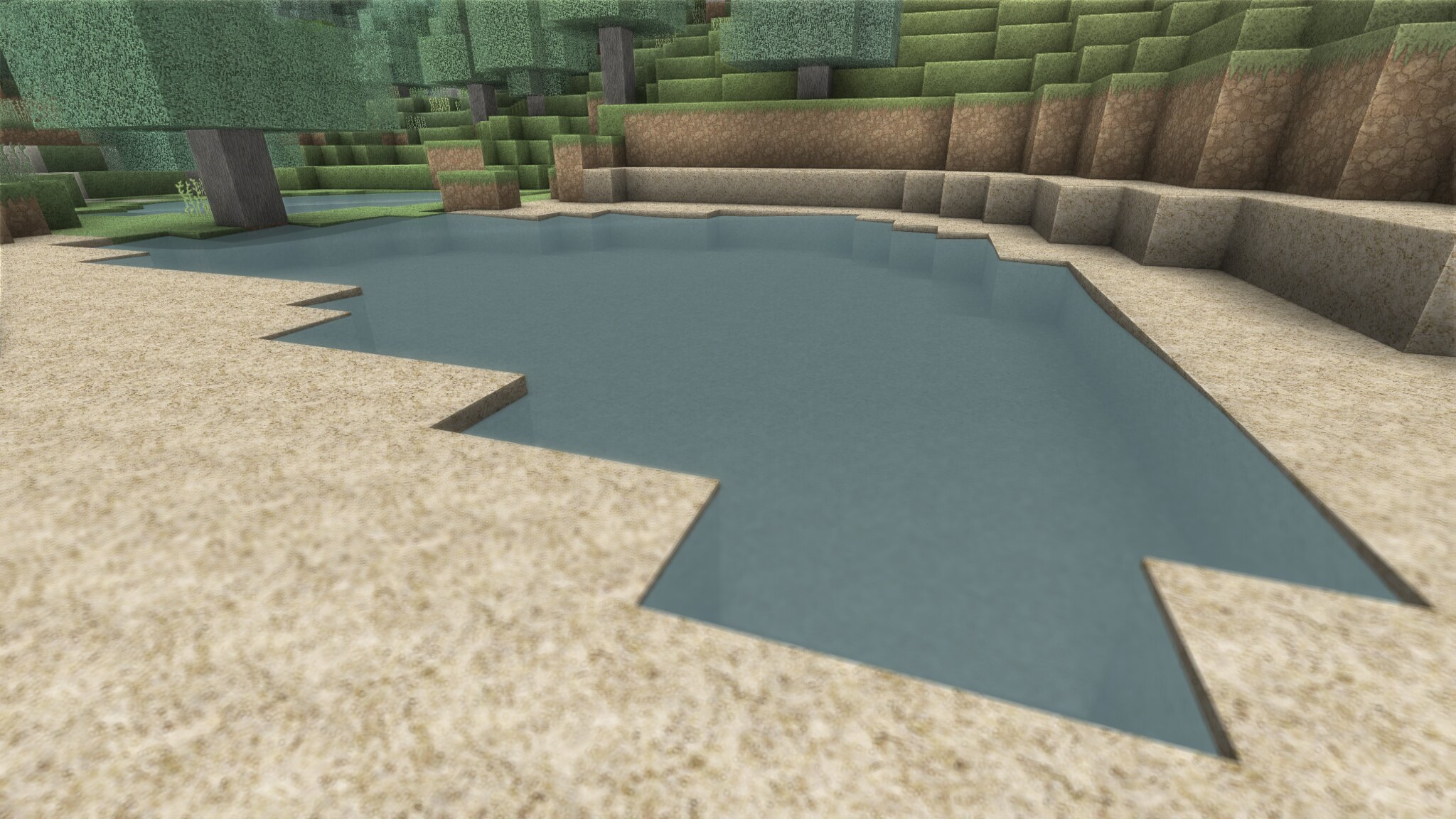The image depicts an architecturally stylized terrace scene, characterized by distinct geometric patterns composed entirely of cubes and rectangles. The foreground features a striking, irregular, and pointed shape in a shade of air force blue, adding a dynamic element to the composition. Behind this structure, there are seating arrangements suggesting a communal or relaxing space. The upper terraces are highlighted in green, possibly indicating designated areas for plants or greenery, creating a contrast with the predominantly angular design. The background showcases a fence and additional green zones, enhancing the visual depth and complexity of the scene.